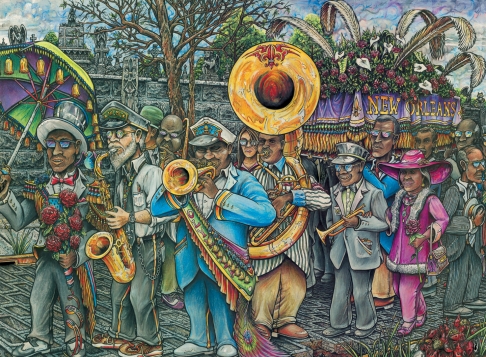This detailed illustration, rendered in a vibrant cartoon-like style, depicts a lively parade in New Orleans. The scene is bustling with a diverse group of people, most of whom are dressed in formal attire such as suits, bow ties, and hats, and many are wearing sunglasses. Leading the parade is an African American man adorned in a black top hat, glasses, a black tuxedo with a red bow tie, and holding a bouquet of red roses in his left hand. Beside him, a white man is playing a blue saxophone and wearing a blue police cap, a white button-up shirt, and a patterned dark tie. Next to them, another man, dressed in a powder blue suit with colorful sashes, is playing a trumpet. Behind him, a man plays a large golden tuba or brass instrument. The parade continues with various participants, including a man with a trumpet, also in a hat and sunglasses, and a woman donning a pink suit and a large pink hat. The backdrop features a float embellished with feathers and flowers that prominently displays the words "New Orleans," along with a cityscape and a large bare tree, completing this festive and colorful depiction of a New Orleans celebration.